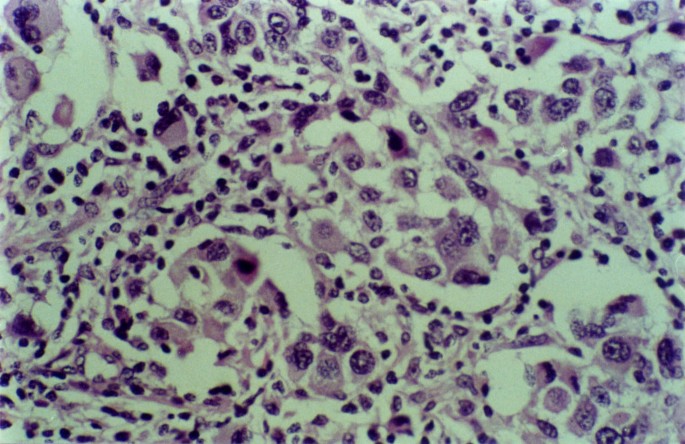The image is a close-up, rectangular photograph, approximately six inches wide and three inches high, with a background of dimmed or shaded grayish-green. The foreground is dominated by swirls and blobby masses of brownish-purple and blue hues, interspersed with tan and brown dots. These dots often have lighter interiors with vein-like spokes radiating outwards, giving the impression of cellular structures under a microscope. Some areas exhibit a bleeding effect where the colors fade into the greenish background. The overall pattern is asymmetrical and chaotic, resembling stained organic material with various imperfect circles and blobs, evoking the appearance of cells or microscopic organisms suspended in a semi-viscous medium.